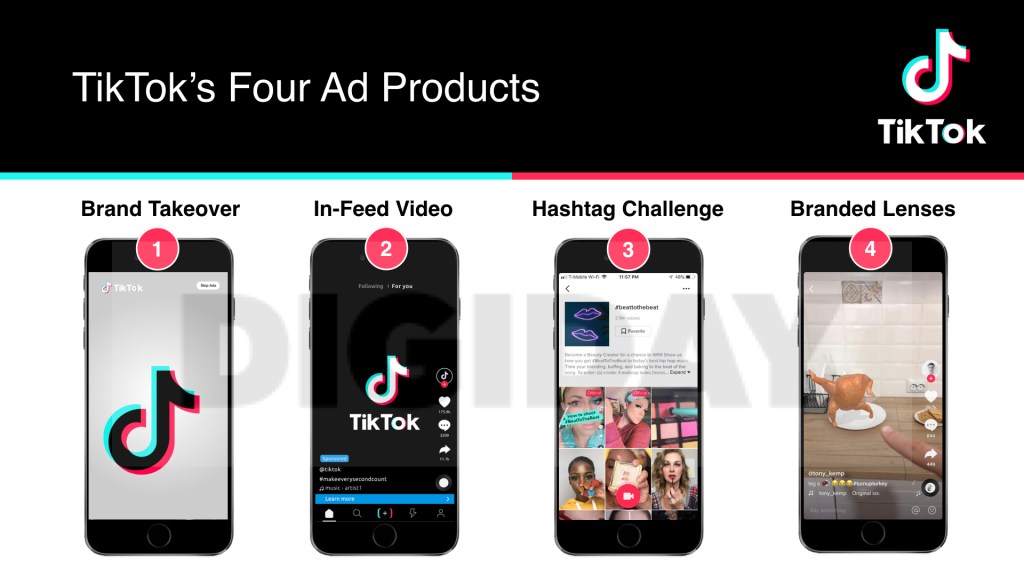This detailed infographic related to TikTok features a prominent black banner at the top with white text stating "TikTok's Ad Products" and includes the iconic TikTok logo—a modified music note with a shimmering green and pink design. Below this banner, intersecting teal and pink lines lead to a white background, which is overlaid with a watermark reading "DIGIDAY."

The infographic is organized into four distinct sections, each denoted by a black cell phone and a pink circle with white numbering.

1. **Brand Takeover:** The first phone displays a simulated TikTok screen with a gray background, showcasing the TikTok logo and a white box with black text.
   
2. **InFeed Video:** The second phone, marked by a pink circle with the number two, shows a black background and multiple icons such as the TikTok logo, a heart, a text bubble, and an arrow. Additional icons at the bottom of the screen include a house, magnifying glass, a plus sign with pink and blue hues, a lightning bolt, and an outline of a person. There are also blue boxes with white text interspersed throughout the interface.

3. **Hashtag Challenge:** The third phone, labeled with a pink circle and the number three, displays a white background with graphic elements that include navy and purple lips, black text, and what appears to be a detailed paragraph. This section highlights various images of real people, primarily women applying makeup. One woman is seen in a pink shirt applying eyeshadow with a palette featuring shades of pink, while another darker-skinned woman holds a makeup product. Additionally, there is a Caucasian woman applying lipstick. Other elements include a teal background, a pink circle with a white camera icon, and visual depictions emphasizing beauty and makeup.

4. **Branded Lenses:** The fourth phone, identified by a pink circle with the number four, features a dancing turkey on a white plate set against a tan countertop and white backsplash. The screen shows icons including a person, a heart, a text bubble, and an arrow, accompanied by some white text.

This infographic succinctly encapsulates the four primary ad products offered by TikTok through engaging visuals and clear labeling.